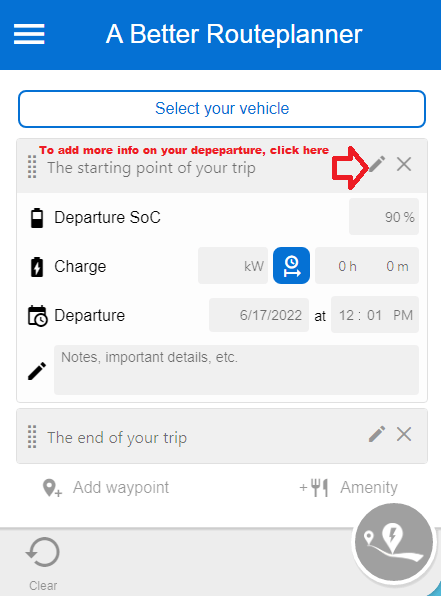This image showcases the interface of a better route planner application. The top center prominently displays the title "A Better Route Planner" in white font within a blue rectangular box that spans the width of the image. To the left of the title, there are three horizontal lines stacked vertically, indicating a menu option, with the entire header left-center justified.

Below the blue bar is a blank space, followed by a white button outlined in blue and featuring blue text that reads "Select Your Vehicle." 

Continuing downward, there is a gray block section labeled with the starting point of the trip. Within this gray section, red text instructs the user to "Add more info on your departure by clicking here." Below the text is a red arrow pointing to the right towards a gray pencil icon next to a gray 'X' symbol, indicating options for editing or deleting the starting point information.